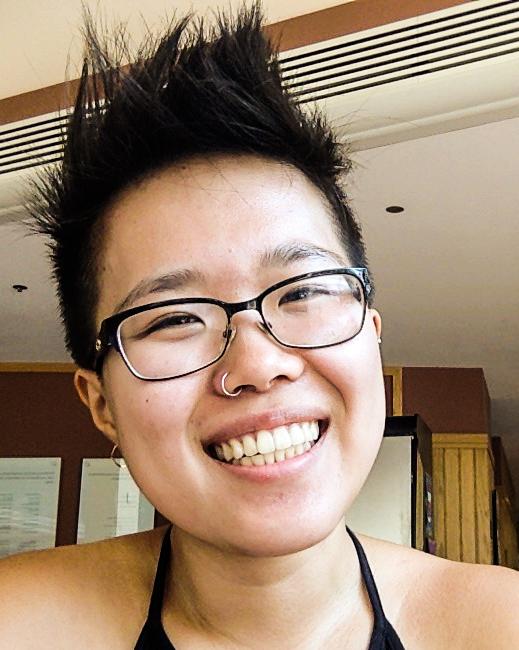This low-resolution photograph features a cheerful young Asian woman with an exuberant expression, showcasing her very white, straight teeth. She is wearing black-framed glasses, a nose ring in her right nostril, and an earring in her right ear; her left ear is not fully visible. Her short, spiky black hair is styled upwards, adding a funky flair to her appearance. She is dressed in a black halter-style top, exposing her bare shoulders. The background suggests she is indoors, possibly in a home or an office setting, with wood paneling on the walls, a white ceiling, and visible lighting fixtures. The overall ambiance of the photo is enhanced by her large, happy smile, making her appear very joyful.